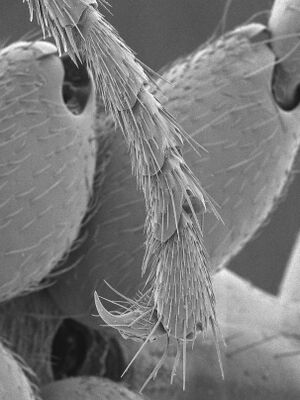This black-and-white photograph, in portrait orientation, presents an extreme magnification of an insect leg, likely that of a mite. The leg's thin, elongated structure is segmented, with the upper portions prominently spanning from the bottom left to the top right. These segments exhibit a cracked texture, similar to human skin viewed up close, and are adorned with thin, wiry hairs that appear almost furry. White hair-like structures densely cover the leg, contributing to its coarse appearance. Toward the top left of the image, a lower leg segment emerges, curving toward the center before bending back under near the bottom, where a small, sharply pointed claw is visible. The background is a dark gray, enhancing the contrast and detail of the leg's surface and its various hair structures. The photograph's realism captures the intricate details, emphasizing the textured, segmented, and spiky aspects of the leg, creating a visually compelling representation of the microscopic world.